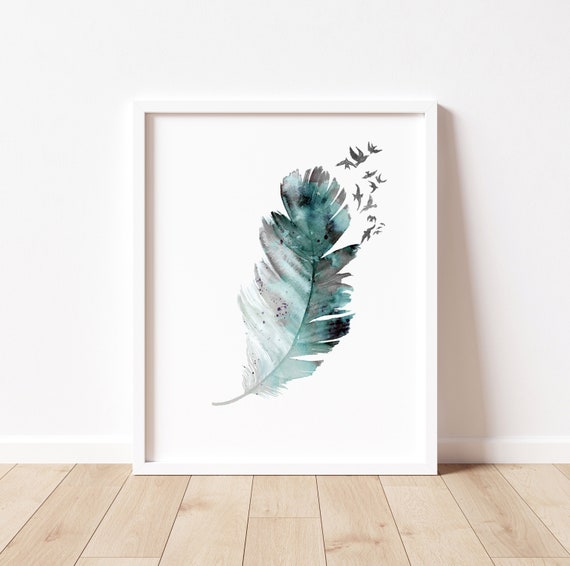In the image, there is a painting propped against a white wall on a pale wooden floor, with vertical wood grain boards. The painting is encased in a white frame and features a white background. The central element is a tall feather standing upright on its quill. The feather transitions in color from white at its base to shades of green, turquoise, blue, and black with hints of brown. From the top right of the feather, about 10 to 15 small birds, colored similarly to the feather, appear to be flying upwards and to the right, creating an impression that the feather is giving rise to these birds. A shadow of the painting can be seen cast on the white wall to the right. The bottom of the wall has white molding, seamlessly blending with the overall light and airy aesthetic.